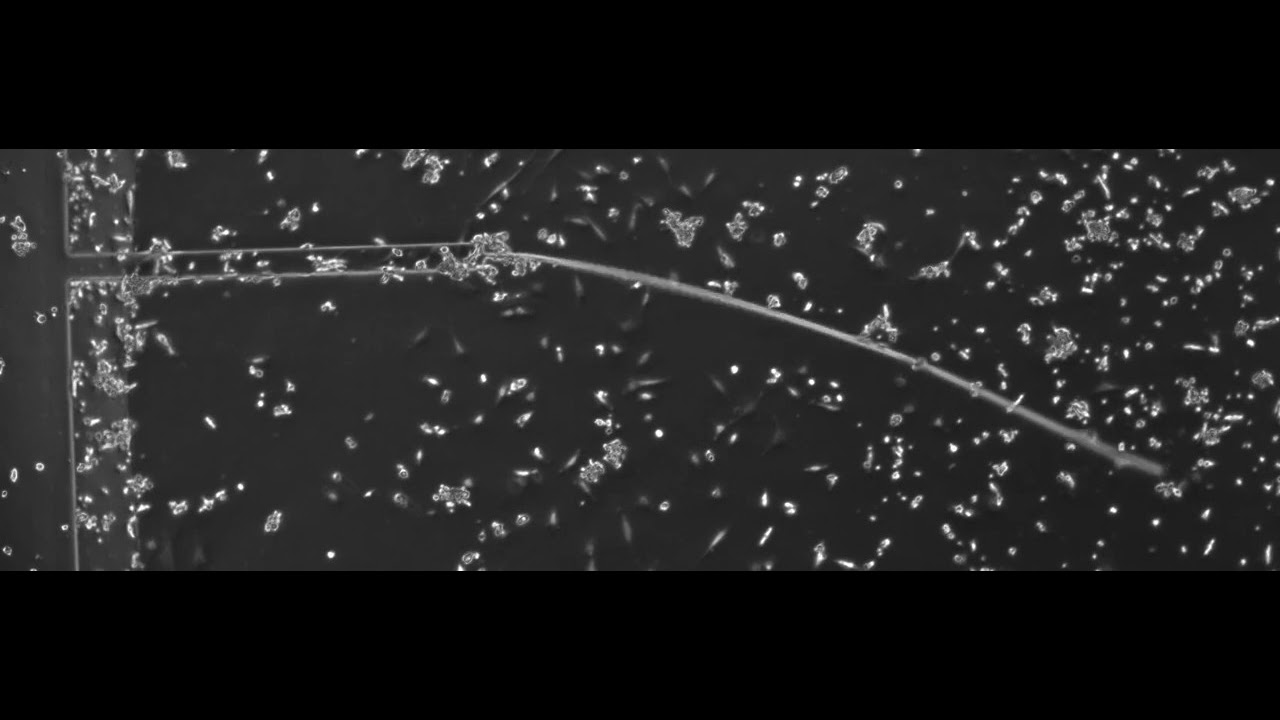This black and white close-up photo captures a highly detailed view of what appears to be seeds flying through the air, reminiscent of the fluffy seeds from dandelions blown in a field. The image is letterboxed with black borders at the top and bottom, framing the central visual content. In the middle, a thin, slightly curved stem forks into two smaller stems towards the top, anchoring the image. From this stem, numerous silver or white oblong seeds, sharply pointed on one end, disperse through the air. 

The seeds are densely packed near the stem, especially towards the right side of the image, giving a sense of motion as they spread out. Some seeds are closer to the background, appearing more grayed out, while others in the foreground are flecked and more pronounced, almost resembling broken glass fragments. Adding to the dynamic composition, there are wispy lines and bubbles overlaying each other, creating an intricate texture. The seeds scatter from left to right, becoming sparser but maintaining a heavy cluster towards the left, suggesting a deceleration as they traverse. The background features additional seeds, subtly blurred to enhance depth. The photo's meticulous detail offers a captivating glimpse into what could be a microscopic view or a staged experimental setup.